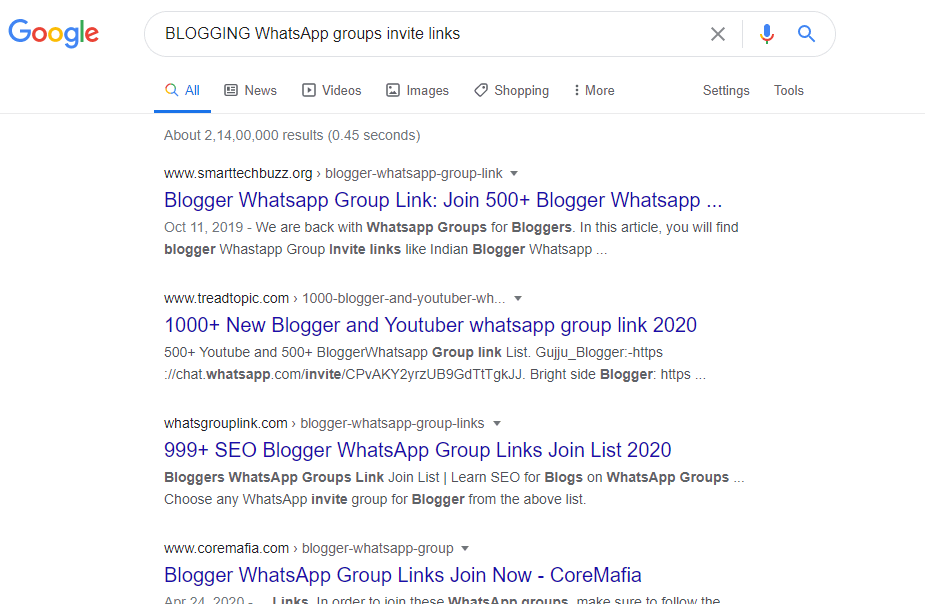The image is a Google search results page focused on "BLOGGING WHATSAPP GROUP INVITE LINKS." At the top left, the iconic Google logo is prominently displayed. Below it, the search bar clearly shows the query in uppercase letters: "BLOGGING WHATSAPP GROUP INVITE LINKS."

The first result leads to SmartTechBuzz.org, highlighted in blue with the title, "Blogger WhatsApp Group Link – Join 500+ Blogger WhatsApp." This is followed by a snippet in gray text dating back to October 11, 2019, mentioning, "We are back with WhatsApp groups for bloggers. In this article, you will find blogger WhatsApp group invite links like Indian blogger..."

Next, the second result is from TrendTopic.com, titled "1000+ New Blogger and YouTuber WhatsApp Group Links 2020." The accompanying gray text elaborates, "500+ YouTube and 500+ Blogger WhatsApp group link list, Guizhou blogger," followed by a long and complex URL.

The third entry points to WhatsGroupLink.com with the title, "999+ SEO Blogger WhatsApp Group Links Join List 2020." Its summary reads, "Bloggers WhatsApp Group Link, Join List, Learn SEO for Blogs on WhatsApp Groups, choose any WhatsApp invite group for blogger from the above list."

Finally, the fourth result is from CoreMafia.com, stated simply in blue as, "Blogger WhatsApp Group Links Join Now CoreMafia."

Each result is distinctly marked with blue titles and gray text descriptions, offering an array of options for bloggers seeking WhatsApp group invites.